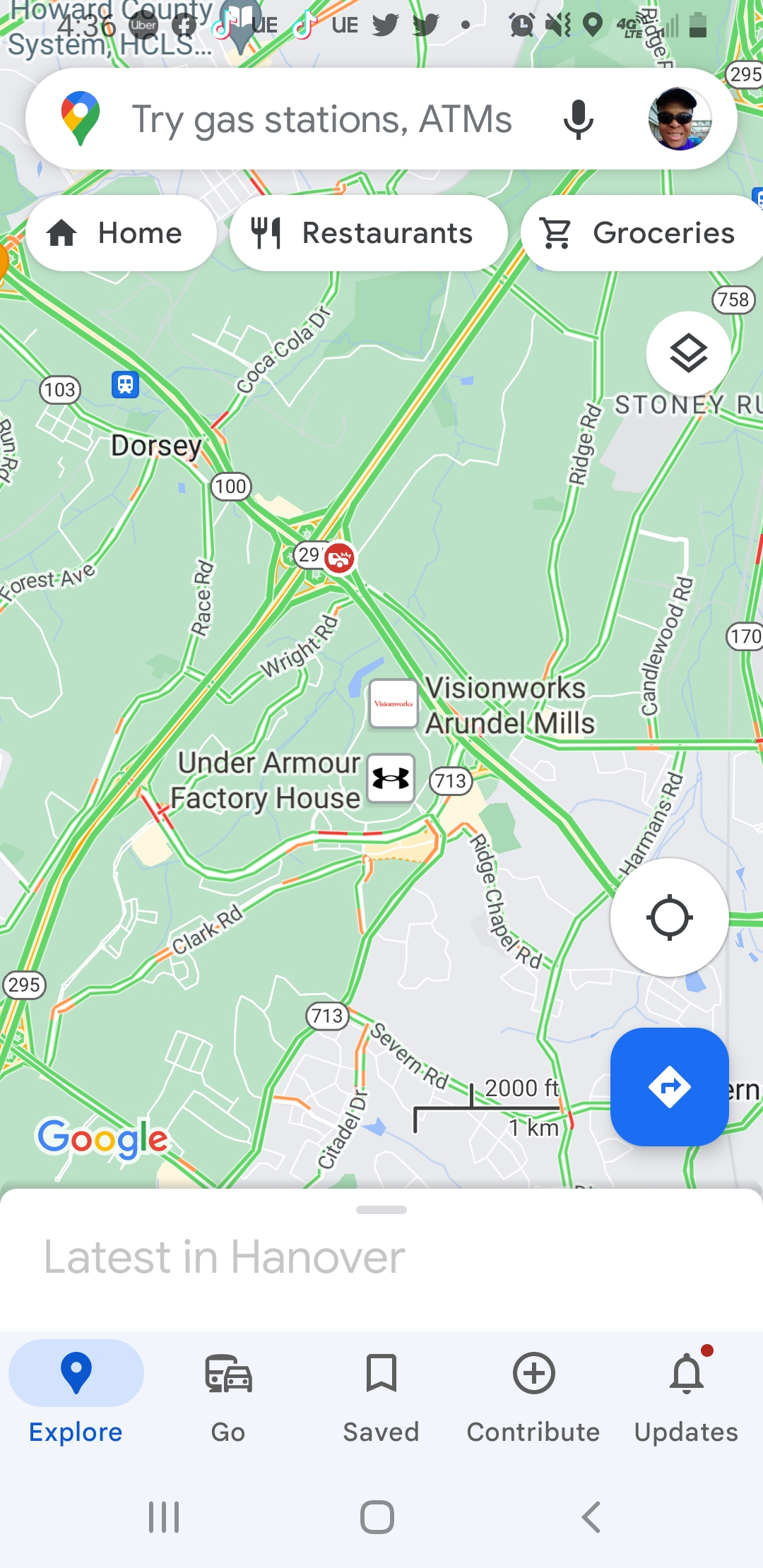The image displays a close-up view of a cell phone screen featuring a Google Maps application. At the top of the screen are various status icons, including those for notifications and active background apps, with some depicting birds. The map highlights an area around the intersection of Highway 29 and Highway 100 near a location referred to as Dorsey. Nearby landmarks visible on the map include VisionWorks, Arundel Mills, Under Armour Factory House, and Highway 713.

Additional routes and landmarks displayed include Ridge Road, Candlewood Road, Stonehenge Drive, Copacabana Drive, Grace Road, Wright Road, Clark Road, and Highway 295. At the bottom left corner, the Google Maps watermark is visible alongside a distance gauge indicating 2,000 feet or 1 kilometer. The interface includes icons for Home, Restaurants, Groceries, and a search bar featuring an icon to search for ATMs and a microphone for voice search. In the top right corner, a small profile picture of the phone’s owner is displayed. The color scheme consists primarily of green and gray, supplemented by Google's signature colors: blue, red, yellow, and green.